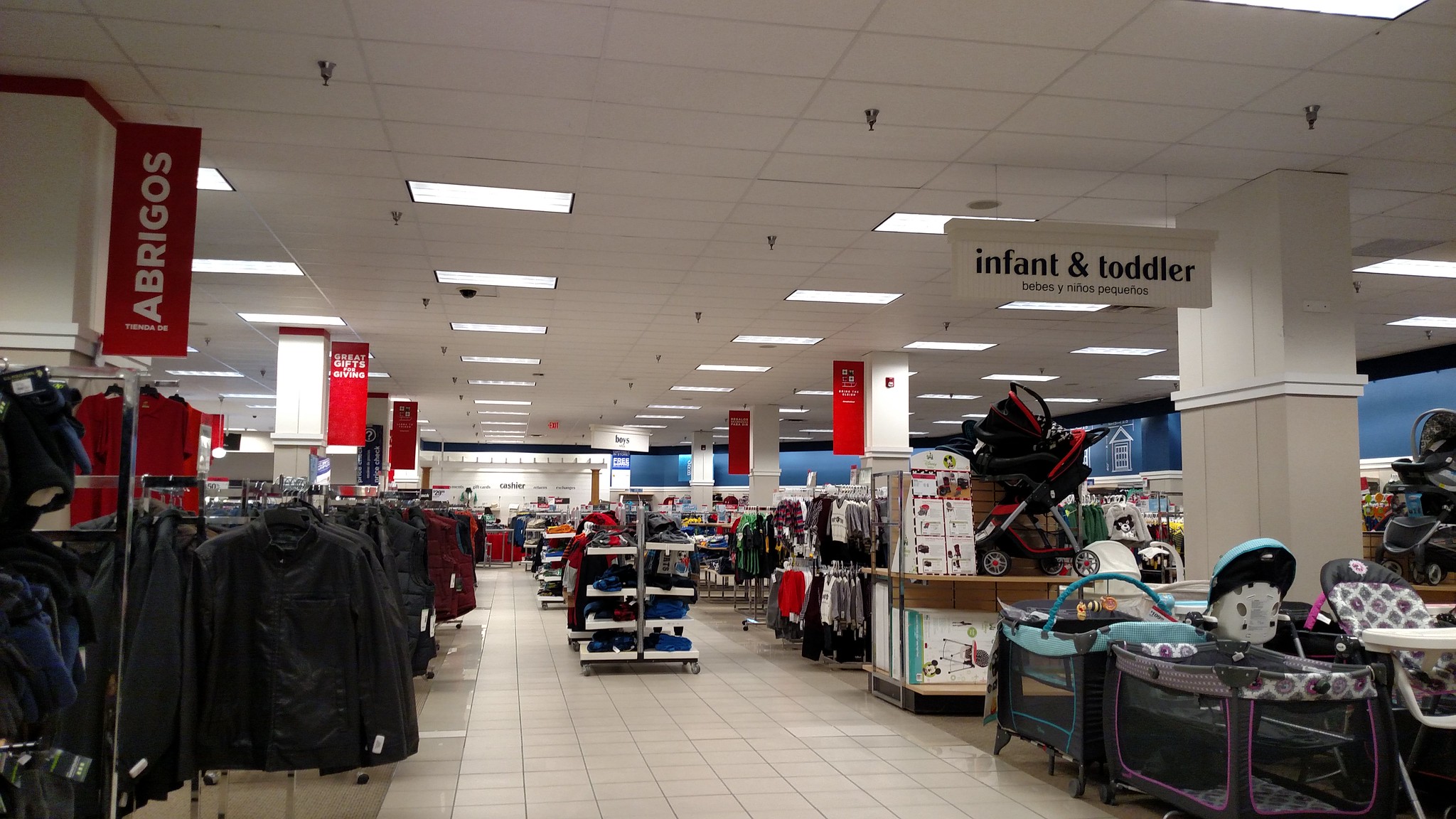The image depicts the interior of a department store. The right side prominently features an "Infant and Toddler" section, marked by a bilingual sign in both English and Spanish, indicating the store may be in a Spanish-speaking location. This section is stocked with various baby-related items, including small clothing, strollers, and baby beds. On the left side of the image, there are racks filled with adult-sized clothing, such as coats and gloves. Additionally, several red signs are visible throughout. In the background, the cashier section can be seen, completing the store's layout.